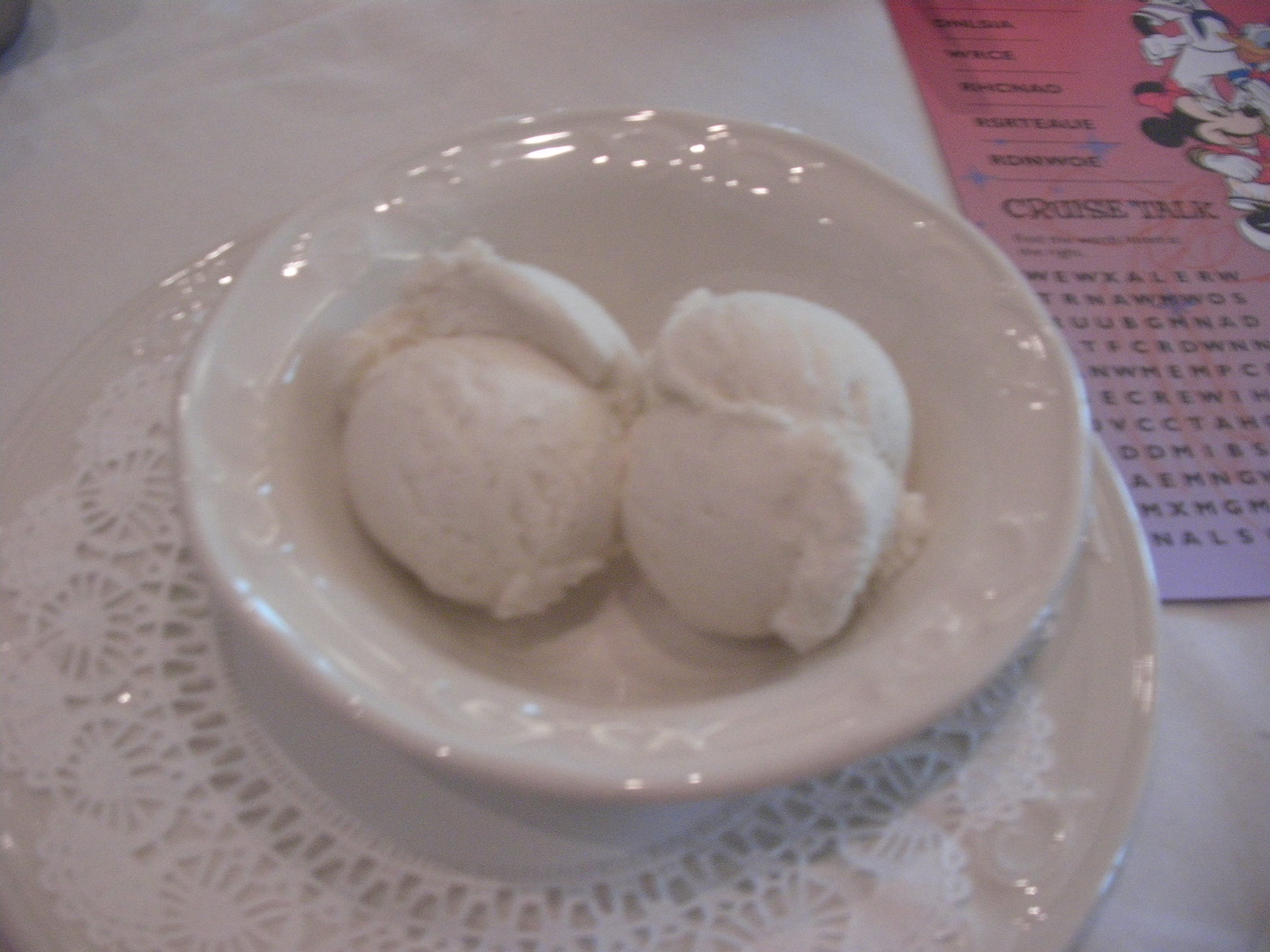In the photograph, there is a white setting featuring two round scoops of vanilla ice cream placed in a white bowl situated on a white plate adorned with a doily. This plate rests on a white tablecloth, creating a clean and minimalist background. In the top right corner of the image, a piece of paper colored in pink and purple is visible. This appears to be a kid-friendly word puzzle featuring Disney characters such as Mickey Mouse, Donald Duck, and Minnie Mouse, with several letters forming part of the game at the bottom left of the paper. The partial view of a spoon is seen at the top edge, partially cut off by the photograph's boundaries, suggesting a casual dining setting.